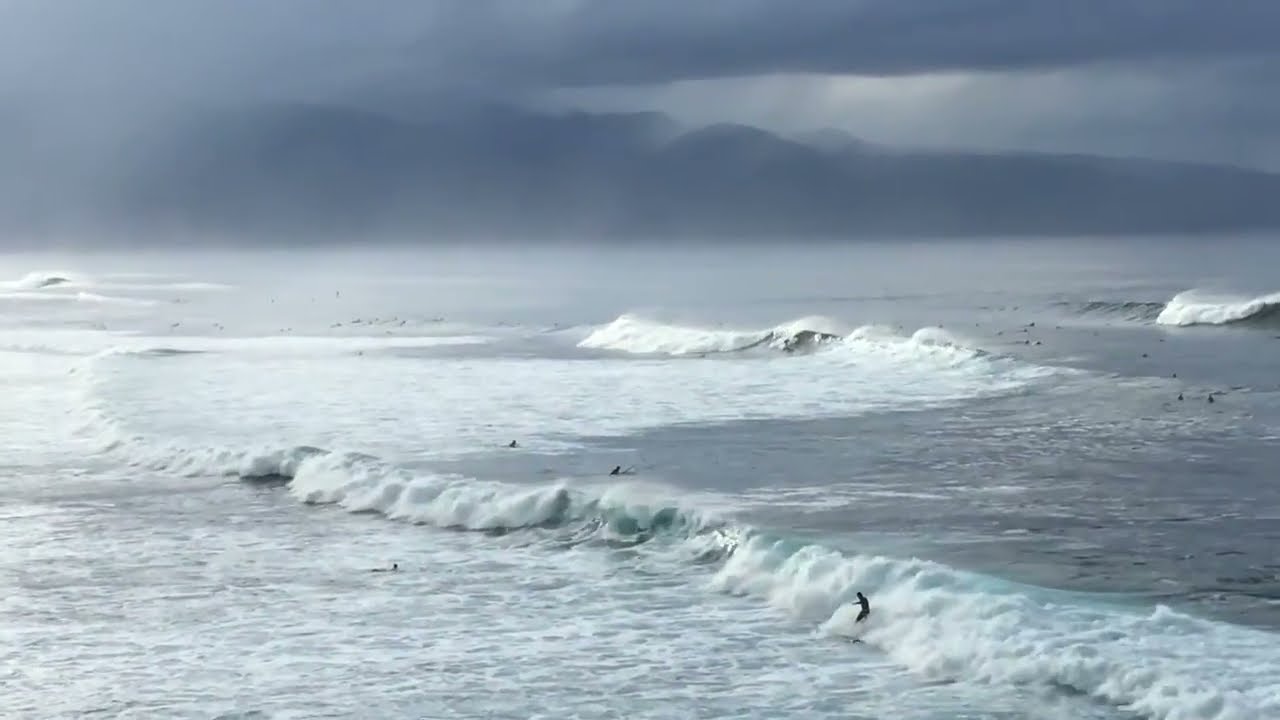The image captures a vast ocean scene dominated by a dramatic grey and blue sky heavily covered in clouds, giving the impression of an approaching storm. The ocean spans the bottom two-thirds of the frame, with the horizon blending seamlessly into the dark, moody sky above. The water moves rhythmically from right to left, punctuated by three distinct sets of white-capped waves rolling in. Alongside these waves, various surfers in silhouette dot the ocean, their tiny forms giving scale to the expansive scene. Some surfers ride the waves while others bob in the water, their identities obscured by distance. In the sky, alternating bands of light and darker shades create a striking contrast, enhancing the overall grey-blue color scheme that unifies the sky and sea.